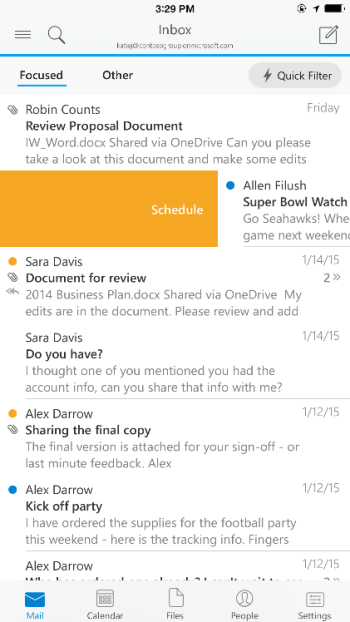The image depicts an email inbox, likely viewed on a smartphone due to its vertically rectangular shape. At the top of the screen, the current time is displayed along with the battery status located in the upper right-hand corner. The word "Inbox" is prominently featured, with tabs labeled "Focused," "Other," and "Quick Filter" just below it.

The inbox shows a series of emails, starting with one from Robin Counts titled "Review Proposal Document," which appears to be linked to OneDrive. Following that is an email from Alan Flush with the subject "Super Bowl Watch - Go Seahawks!" highlighted by an orange schedule bar, indicating that the email might have been selected. 

Further down, multiple emails from Sarah Davis are listed: one requesting a document for review, another asking "Do you have the account info? Can you share that info with me?" Additionally, two emails from Alex Darrell follow, with subjects "Sharing the Final Copy" and "Kickoff Party - I've ordered the supplies for a football party this weekend," respectively, suggesting a blend of professional and personal correspondence, possibly relating to workplace activities and Super Bowl party planning. 

The timestamps on the emails suggest dates around January 12 and January 14, 2015, and the current time displayed on the phone is 3:29 PM. The exact date when the picture was taken is not visible from the image, but it provides a snapshot of someone's email communications during that period.